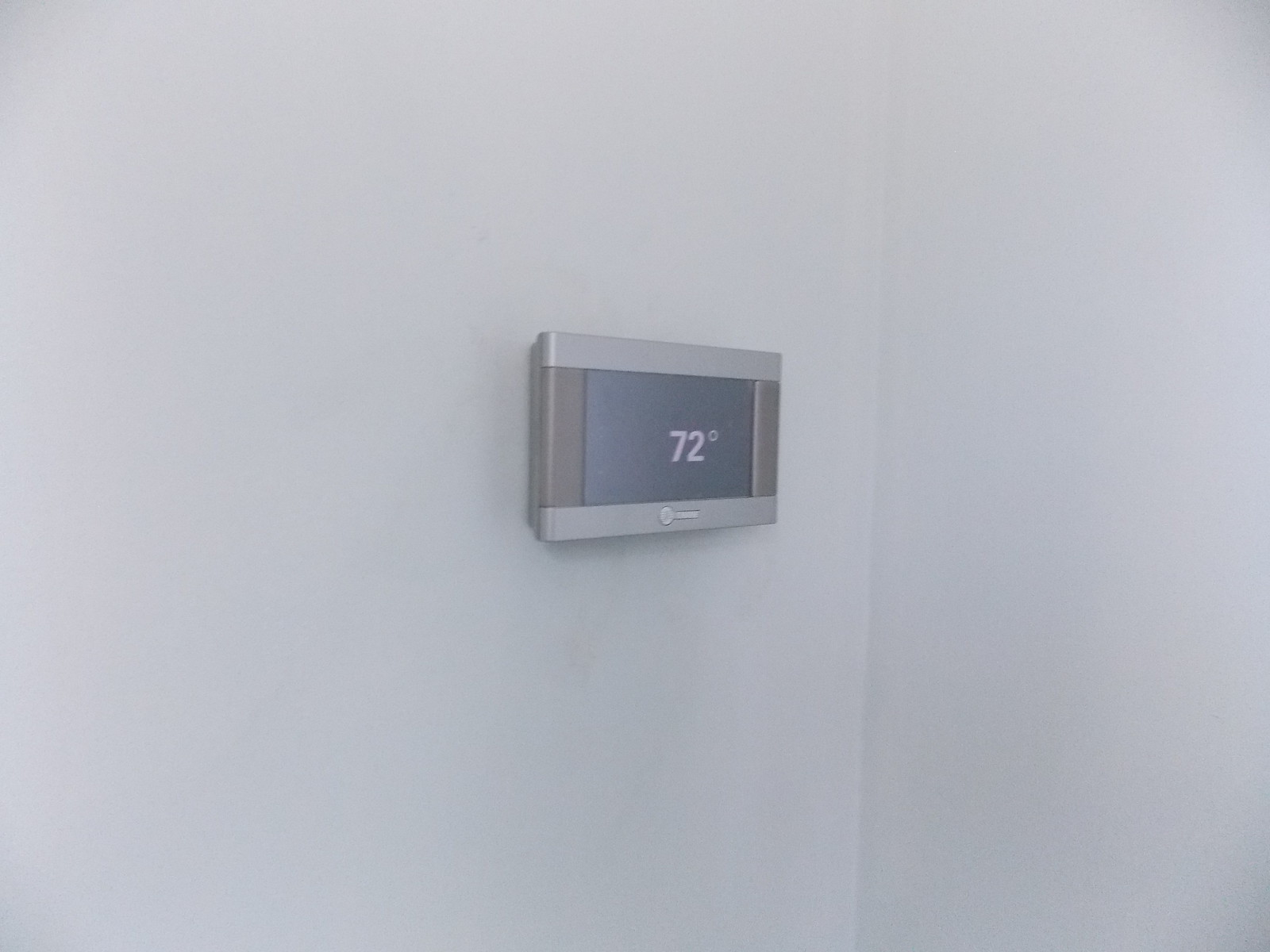The image features a predominantly white wall that is intersected by a vertical seam slightly to the right of the center, indicating the corner where two walls meet. On the left side of this seam, there is a modern air conditioning thermostat. The thermostat is rectangular in shape, with horizontal gray-silver sections at both the top and bottom, likely made of plastic. In between, there are two vertical brown elements running parallel from top to bottom. The brand name on the bottom gray section appears in white but is illegible. The central portion of the thermostat is black, prominently displaying "72 degrees" in white text. A subtle shadow is cast below the thermostat, adding depth to the scene against the otherwise plain wall.